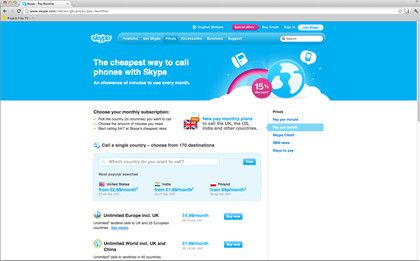This is a screenshot of a website, likely a homepage, displayed in landscape orientation, being slightly wider than it is tall. At the very top of the page is a gray bar housing an open tab featuring a blue icon and black font.

Below this, a larger gray bar spans horizontally across the screen, containing a back arrow, a home icon, a refresh button, and a white search bar with black text inside. Beneath this bar, another gray section features an orange icon on the left, potentially indicating a frequently visited site.

The next segment is a long horizontal bar with a blue background. Centrally placed on this bar is a logo resembling the Skype logo, characterized by blue letters with a white border. Adjacent to this logo is a blue oval-shaped menu bar with white font and another white search bar underneath.

Directly below this blue section, white text proclaims "The cheapest way to call phones with Skype." This text is accompanied by a logo of a planet, several phone icons, and a red or pink circle labeled "15% off" in white font.

Further down the page, a section invites users to "choose your monthly subscription," presenting options and information within a blue bar. Following this, various white areas contain additional links and details, though the small font size makes them difficult to read.